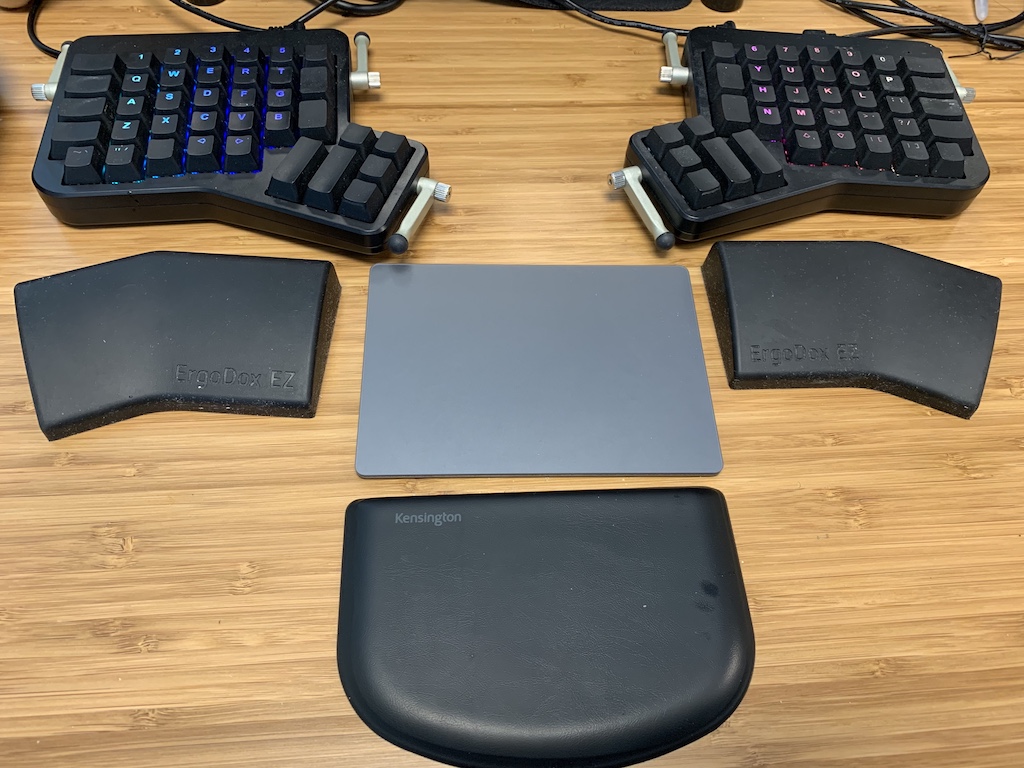The photograph depicts an ergonomic keyboard setup spread across a light brown, wooden desk. This specialized keyboard is visibly split into two halves, designed for ease and flexibility, allowing the user to place one half on the left and the other on the right. Both halves of the keyboard feature black keys with blue LED backlighting on the left side and pink LED backlighting on the right side. The left half includes keys labeled 1-5, QWERT, ASDFG, ZXCVB, while the right half includes keys labeled 6-0, YUIOP, HJKL;, and NM.

Between the two halves lies a gray mouse pad, slightly above the center. Below the mouse pad is a digital mouse tracking pad. Various objects are neatly placed around the keyboard: two black ergonomic wrist guards are located beneath each half of the keyboard, one branded with "ERGO-DEX-EASY" on the left and the other with "ERGO-DEX" on the right. Additionally, a Kensington-branded padded ergonomic wrist rest sits below the mouse pad.

Three silver antennas with black tops are positioned prominently on both halves of the keyboard, suggesting a wireless communication feature. This comprehensive setup, designed for ergonomic comfort, efficiently utilizes the desk space, while the wooden desk's light brown tones provide a pleasant aesthetic contrast to the black and gray components.